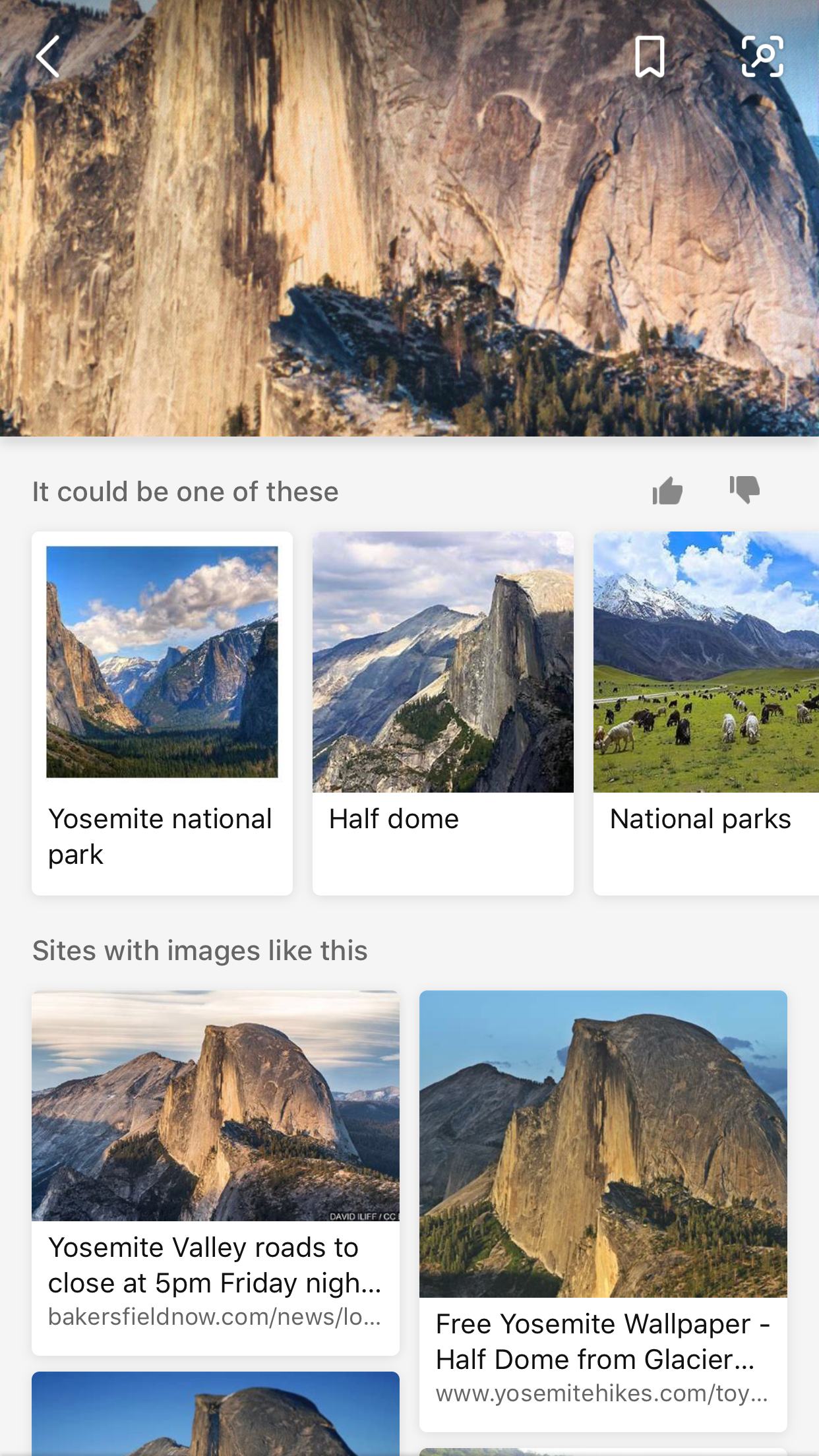The image appears to be a collection of search results, displaying multiple photos resembling the iconic landscapes of Yosemite National Park. The top photograph prominently features the famed Half Dome, a towering granite peak with minimal vegetation, noted for its distinct appearance of a 'half dome.' Below this, additional images suggest variations of similar natural scenery, alongside text references identifying the location as Yosemite. The results also display links with captions such as "Yosemite Valley Road closes at 5 p.m. Friday," "free Yosemite wallpaper," and "Half Dome Glacier Park." Further down, partially visible images depict the breathtaking vistas of Yosemite Valley, showcasing snow-capped peaks, verdant valleys, and possibly cattle grazing in the meadows. The overall presentation strongly indicates that the original image search centered around Yosemite’s majestic Half Dome.